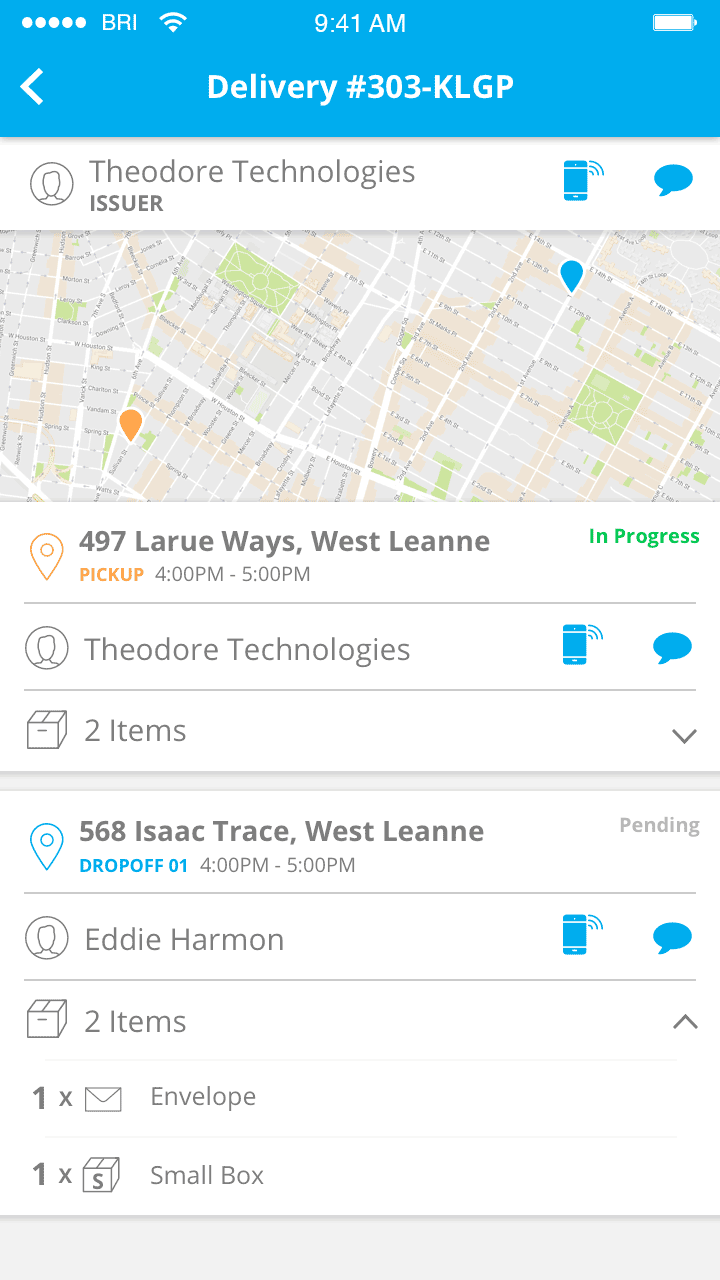The image captures a smartphone screen displaying a delivery tracking app. The time 9:41 AM is prominently shown at the top center, with a full battery icon and strong internet signal bars visible. The screen details the delivery number 303 KLGP, issued by Theodore Technologies. It includes the country of origin and a message notification.

The screen also features a map that likely shows the delivery route. The pickup location is 497 LaRue Ways, West Leanne, with a pickup time window between 4 to 5 PM, and the status is marked as 'In Progress.' Two icons are on the right: one resembling a coffee container (though its purpose is unclear) and a speech bubble icon for messages.

Further down, the screen lists 'Two Items' with a box icon next to it, indicating expandable details that are currently not displayed. The drop-off location is 568 Isaac Trace, West Leanne, also scheduled between 4 to 5 PM and marked as 'Pending.' The recipient is Eddie Harmon. Additional item details show one envelope and one small box.